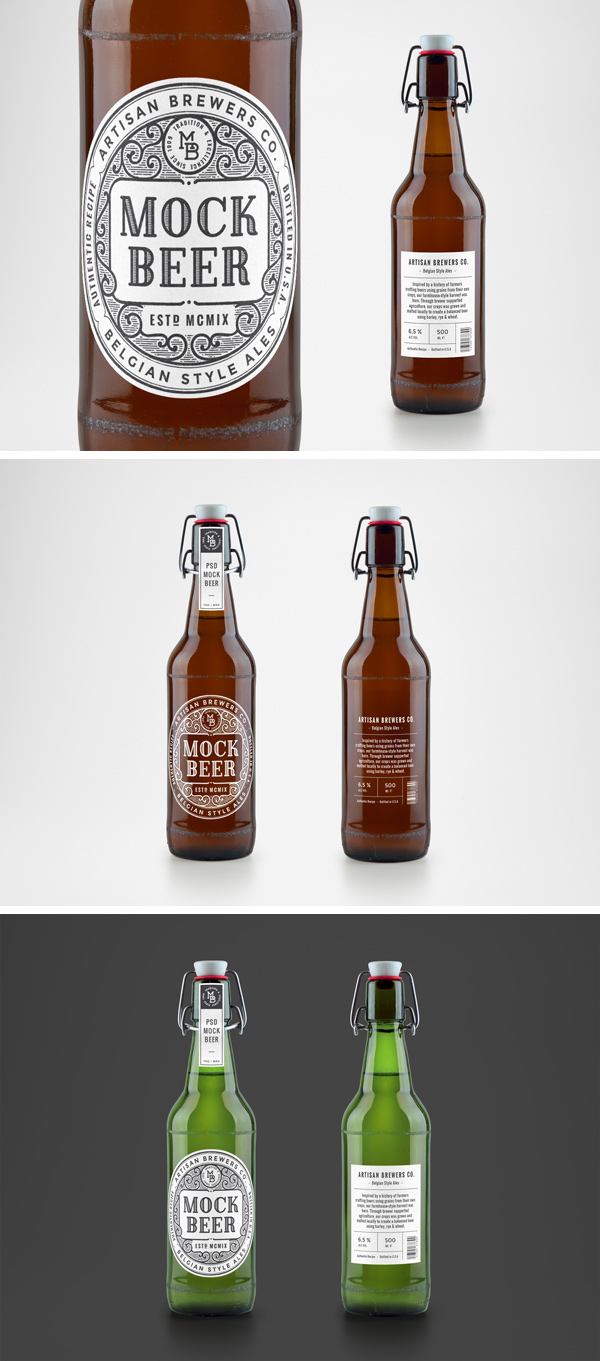The image is a detailed three-part mock-up showing different Belgian-style ale bottles branded as "Mock Beer" by MikMiks, established in 2020. Each mock-up presents a distinct variation of the bottle design on a white and black background. 

The top image features an amber bottle with a white, oval-shaped label. The label includes a decorative swirling pattern and key text: "Mock Beer" in the center, "Artisan Brewers Co." at the top, and "Belgian Style Ale" at the bottom. This bottle also has a Grosch-style pop-off cap. 

The middle image displays a similar amber bottle. However, the text and swirl design appear to be directly imprinted onto the bottle itself, without a distinct label. 

The bottom image showcases a green bottle, which mirrors the design of the first bottle but with a white background label similar to the top image. Thin white lines divide this part of the image, highlighting the green bottle against a contrasting background. 

These mock-ups effectively present different design options for the brand's packaging, each with subtle yet impactful variations.